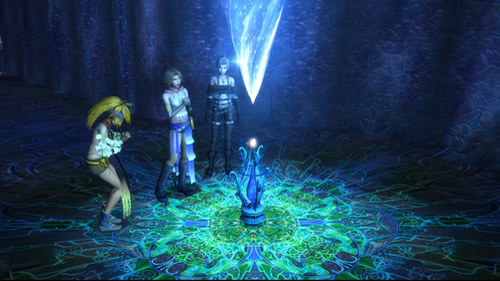The image appears to be from a video game or animated cartoon, illustrated in shades of blue and dark blue. It depicts three characters standing in a dark, cave-like environment with green and blue patterns on the ground reminiscent of peacock feathers. 

In the center of the scene is an object emitting energy, held by a tealish-purple rack or metallic pedestal. Above it, a large, shiny, V-shaped crystal hangs, appearing to draw energy downwards towards the object, which glows as if about to ignite.

The three characters include a blonde girl with a long yellow ponytail who appears to be bound with white tape or rope. She is wearing shorts, exposing bare legs, and tennis shoes. To her right stands another woman in blue pants, and to her right is a third woman dressed in a black ensemble. They seem to be wearing fighter gear or unusual clothing typical of video game characters. The background suggests a dark, mysterious cave setting, enhancing the image's adventurous and mystical atmosphere.